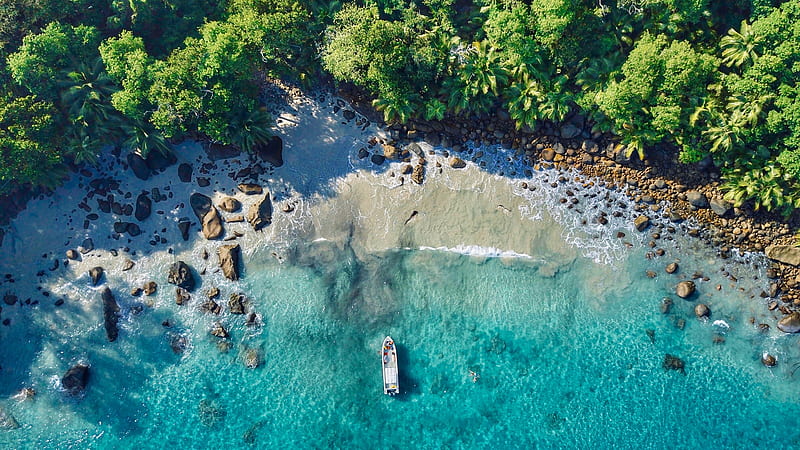The image is a landscape-oriented color photograph captured from a drone, offering a bird's-eye view of a scenic beach. At the bottom half of the image lies a stunningly clear aqua blue ocean, shallow near the shoreline with small white waves crashing gently onto the sand. The beach's white sandy stretch, slightly tinged with gray where the water has touched it, curves gently across the center of the image from left to right. Prominent in the composition is a thin white boat positioned vertically, heading toward the shore, with hints of people visible near its pointed front. Scattered across the beach are several large brown boulders forming a natural outline alongside the sprawling green palm trees and surrounding vegetation at the top of the image. The brown rocks create a noticeable wall-like structure extending from the middle right to the upper back of the scene, adding to the beach’s picturesque setting. The overall photograph captures the vivid colors and detailed textures of a tropical seaside landscape with striking realism.